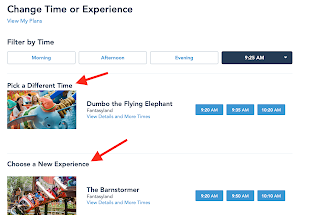This screenshot features a user interface with a clean white background. At the top, in bold black text, it reads "Change time or experience." Directly below this, in smaller blue text, is the link "View My Plans." Following that, another heading in black text states "Filter by Time," introducing a set of four boxes. The first three boxes, labeled "Morning," "Afternoon," and "Evening," are in blue text. The fourth box displays a specific time range.

Underneath these controls, there are two movie selections each accompanied by images: "Dumbo the Flying Elephant" and "The Barnstormer." 

- "Dumbo the Flying Elephant" has a heading in blue text, "Pick a different time," with a red arrow pointing towards it.
- "The Barnstormer" has a heading, also in blue text, saying "Choose a new experience," marked by another red arrow.

A thin gray line separates these two items. For each movie, there are three blue rectangles containing white text with available times listed: "9:20 a.m.," "9:35 a.m.," and "10:20 a.m."

This layout is designed to provide users with clear options for managing their plans and selecting different times for their chosen experiences.